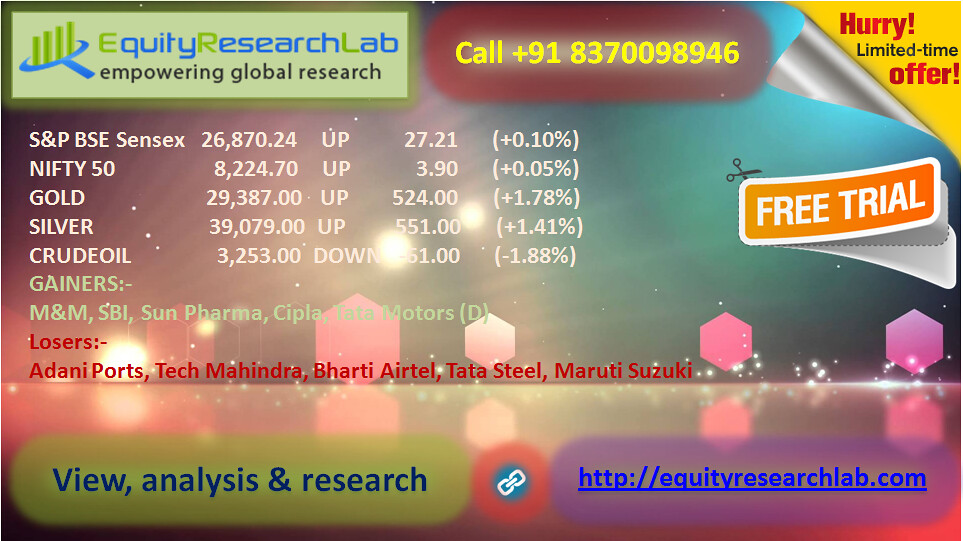The image is an advertisement for Equity Research Lab, a company specializing in global stock research. The design features a prominent logo for Equity Research Lab in the top left, set against a maroon background. The tagline "Empowering Global Research" is displayed within a green-colored rectangle. A yellow triangle in the top right corner announces a "Hurry, Limited Time Offer," with the word "hurry" and "offer" in red font and "limited time" in black. Below this, an orange banner highlights the availability of a "Free Trial," depicted with scissors as if it's a coupon being cut out.

The advertisement includes extensive stock market information. Stock quotes show S&P BSE Sensex at 26870.24, up by 27.21 points (+0.10%), and Nifty 50 also up. Commodities like gold and silver are marked as up, whereas crude oil is down. Listed gainers include M&M, SBI, Sun Pharma, and Tata Motors, while losers feature Adani Ports, Tech Mahindra, Bharti Airtel, Tata Steel, and Maruti Suzuki.

Hexagons are arranged horizontally near the bottom of the image, above a URL ("http://equityresearchlab.com") and a chain template in the bottom right corner. The color palette is vibrant, incorporating shades of blue, green, yellow, red, orange, pink, white, and light blue, adding to the dynamic and eye-catching nature of the advertisement. The phone number to contact the lab, "91-837-009-8946," is also prominently displayed near the top.